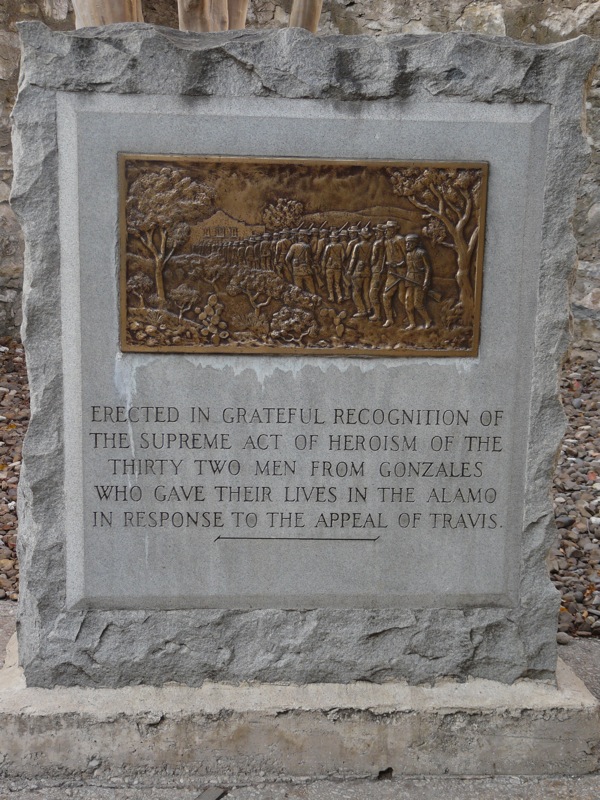The image depicts a stone monument reminiscent of a gravestone, with a rough, chiseled gray stone backdrop and a flat gray central area. This monument, mounted on a cement or marble pedestal, features a prominent bronze plaque in the upper half. The bronze plaque is intricately detailed with a depiction of soldiers marching in a line, holding guns, flanked by trees and vines. Below the bronze image, the stone bears an engraved inscription in capital letters: "Erected in grateful recognition of the supreme act of heroism of the 32 men from Gonzales who gave their lives in the Alamo in response to the appeal of Travis." The text is directly carved into the stone, highlighting the monument's solemn commemoration of these heroic acts.